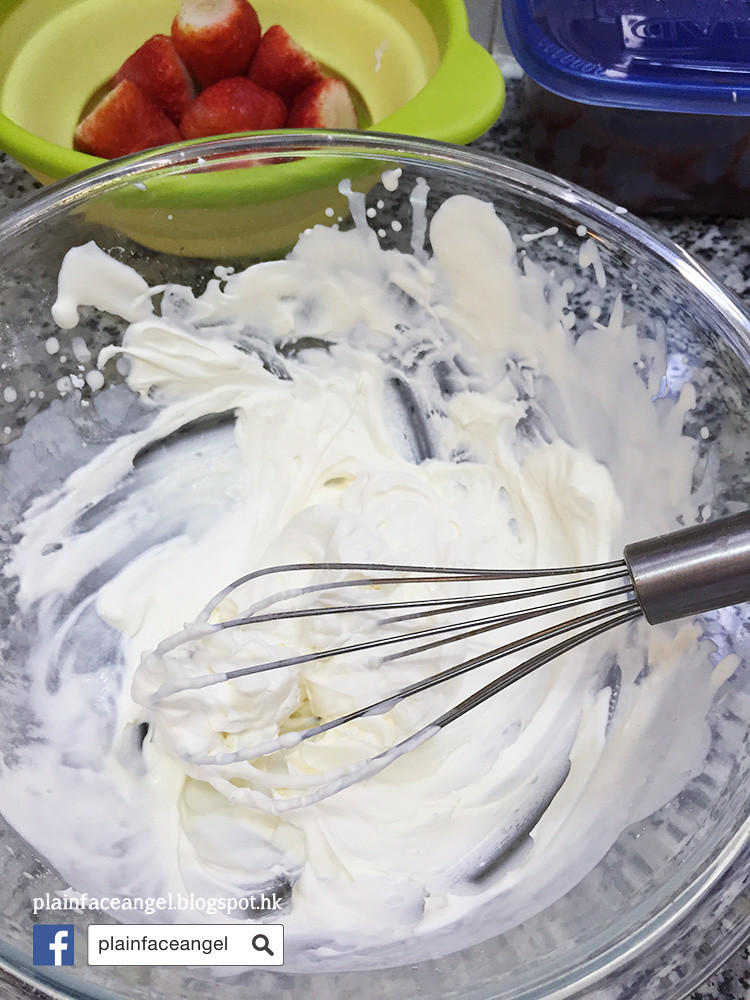The image depicts a food preparation scene on a black and white flecked countertop, which appears to be a stone or marble surface. The central focus is a large clear glass bowl containing a white cream substance being mixed by a silver whisk. Positioned to the upper left is a light green and yellow bowl with red strawberries that have had their tops removed. To the right of the mixing bowl, there is a square but rounded Tupperware container with a clear base and a blue lid. In the bottom left corner of the image, there is an overlay of text and symbols, including the words "plain face angel" in black lowercase print beside a blue Facebook icon, along with "plainfaceangel.blogspot.hk" and a white search bar with a magnifying glass icon.